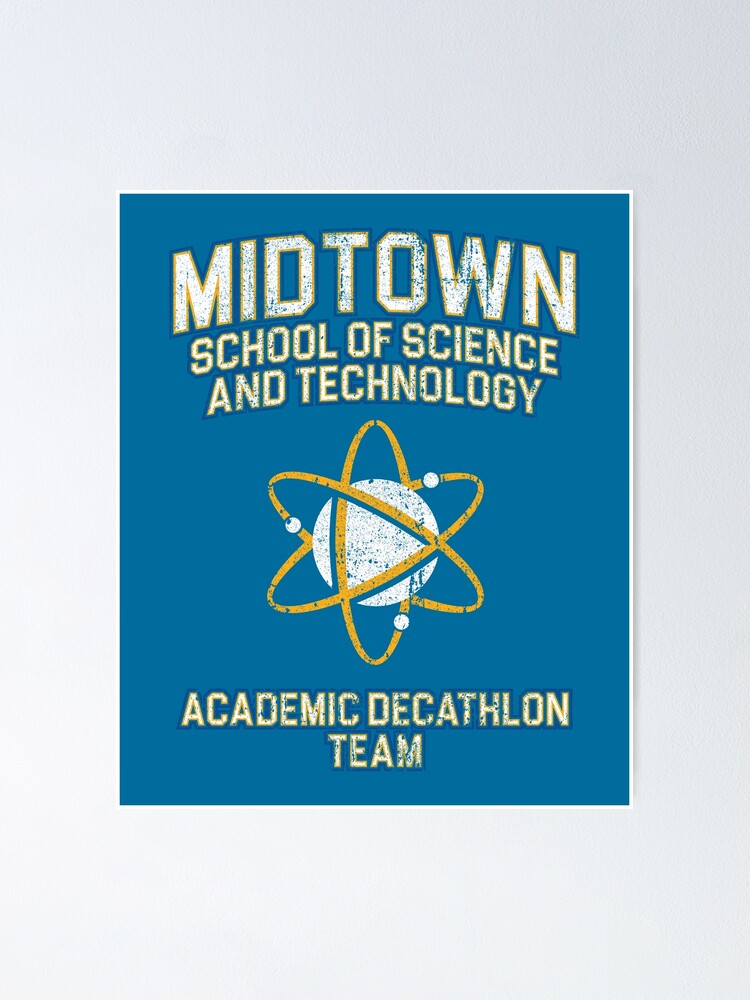This vibrant color illustration, reminiscent of a printmaking piece, is set against a flat gray backdrop and adopts a vertical format. This design utilizes a restrained color palette of yellow, blue, and white to striking effect. 

At the heart of the visual, a round globe-like object is encircled by a spiral star, evoking the imagery of a planet in motion. The composition is anchored by bold block text that reads "Midtown School of Science and Technology, Academic Decathlon Team," appearing both above and below the central logo. The text, featuring a grainy texture that gives it a rubbed-off, volumetric look, adds to the piece's tactile quality.

Additionally, the central image itself also exhibits some deliberate wear, contributing to the overall printmaking aesthetic. The illustration is neatly framed by a thin white border, which further accentuates its presence on the simple, flat blue canvas. This thoughtfully designed piece manages to be both striking and elegant in its execution.